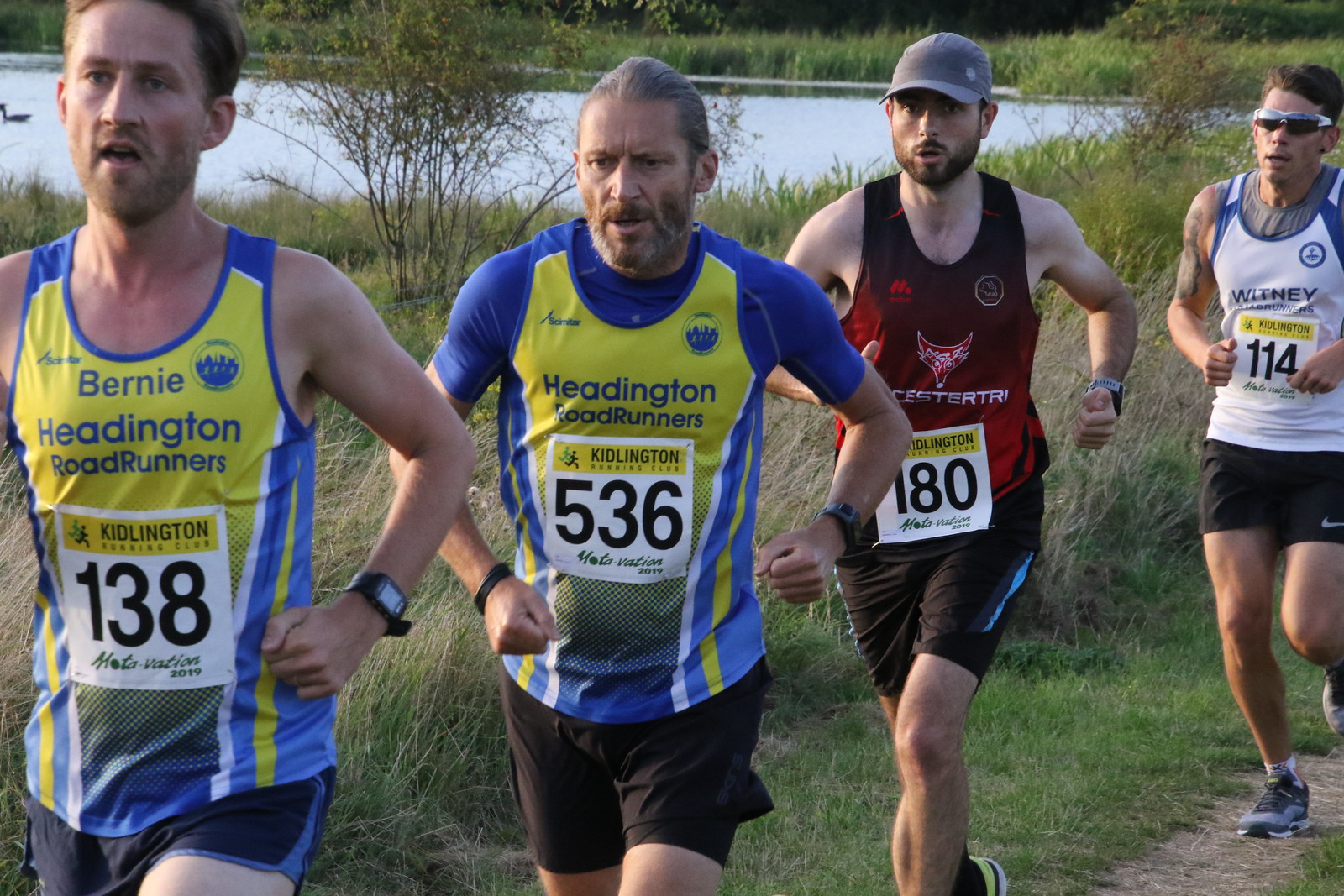In the image, four male runners—each of varying ages—are competing on a light brown dirt track, which has grass growing on either side and extends further into the background. Beyond the track, there is a body of water on the left edge featuring a boat, and surrounding the area are tall shrubs and trees. In the front of the pack is a middle-aged white man with short brown hair and a light beard, wearing a light blue and yellow tank top, blue shorts, and the number 138 on his chest. Next to him is an older white man with gray hair combed back, dressed in a light blue tank top with a yellow panel, black pants, and the number 536 on his shirt. Behind them is a slightly younger white man sporting a gray baseball cap, a dark reddish sleeveless tank top, black pants, and the number 180. The fourth runner is a young white man with sunglasses and a tattoo on his left arm, wearing a white tank top, black pants, and the number 114. The lush scenery of grass, trees, and water frames their path, enhancing the natural beauty of the race setting.